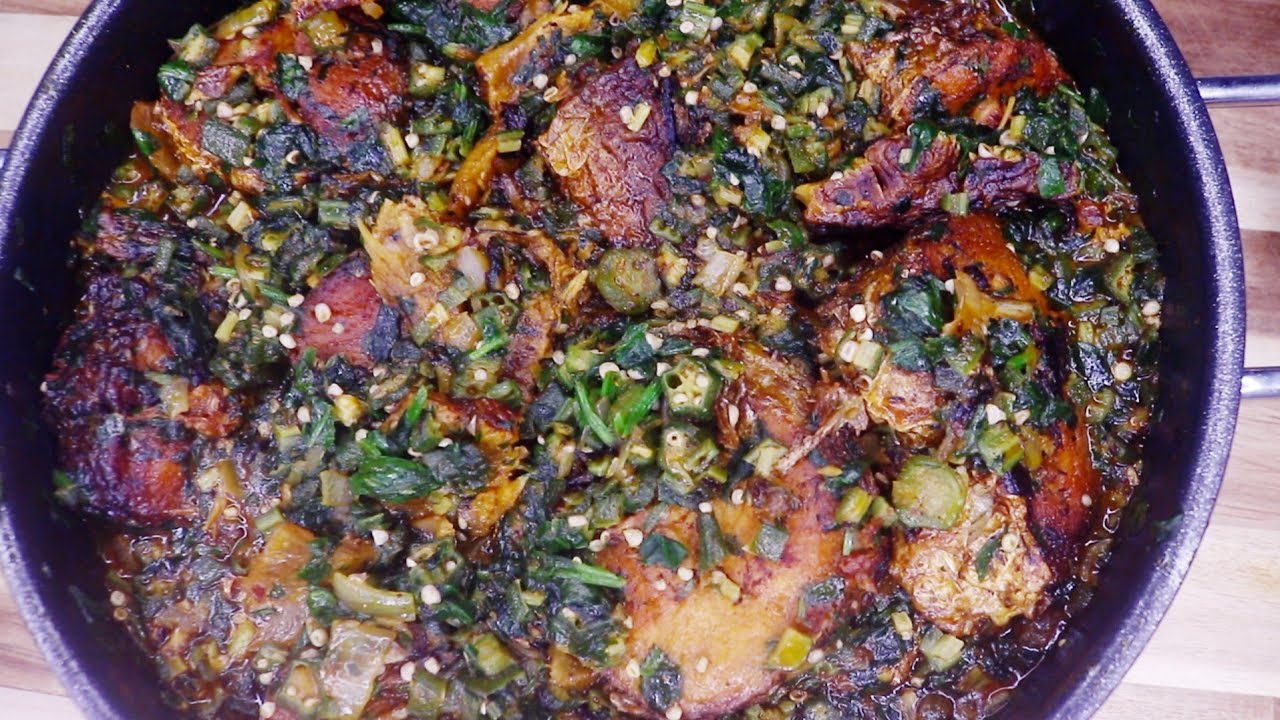This vibrant image showcases a Culinary Supreme dish presented in a large black cast-iron skillet, slightly off-center on a light-grained, brown wooden surface. The skillet, with its handle visible on the right, brims with a colorful array of well-cooked ingredients. Predominantly, there are green, red, and yellow peppers, chopped finely, scattered throughout the dish. Accompanying these are translucent, white onions, green beans, and bright yellow corn kernels. Amongst the vegetables, pieces of richly browned, almost crispy-looking meat, possibly chicken, add a hearty element. The scene suggests a bright and lively kitchen setting, possibly indicative of home cooking or a vibrant culinary display on a cooking show or food website. The image, devoid of any textual elements, springs to life through its varied and vivid colors, ranging from shades of brown and tan to purples, greens, and oranges, enhancing the appetizing and visually appealing nature of the dish.